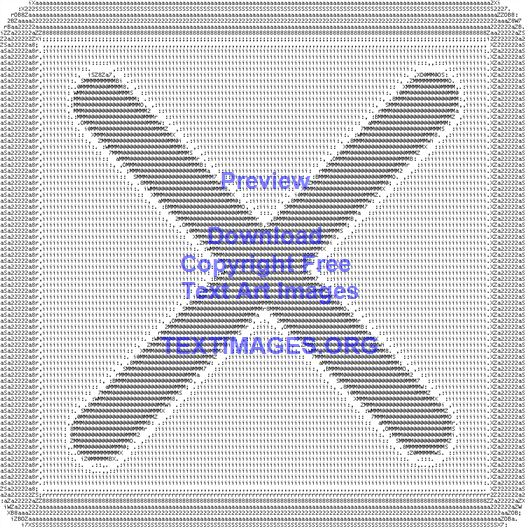The image is a computer-generated square in black and white with a darker black-and-white dot border surrounding the square. Inside, there is a lighter gray interior featuring a large, pixelated X that spans from one edge of the square to the other. In the middle of this X, in purple text, it reads "PREVIEW," followed by "Download Copyright Free Text Art Images" in smaller purple writing below. At the bottom of the image, the text "TextImages.org" is displayed, indicating that this image serves as an advertisement for the website offering downloadable, copyright-free text art images.